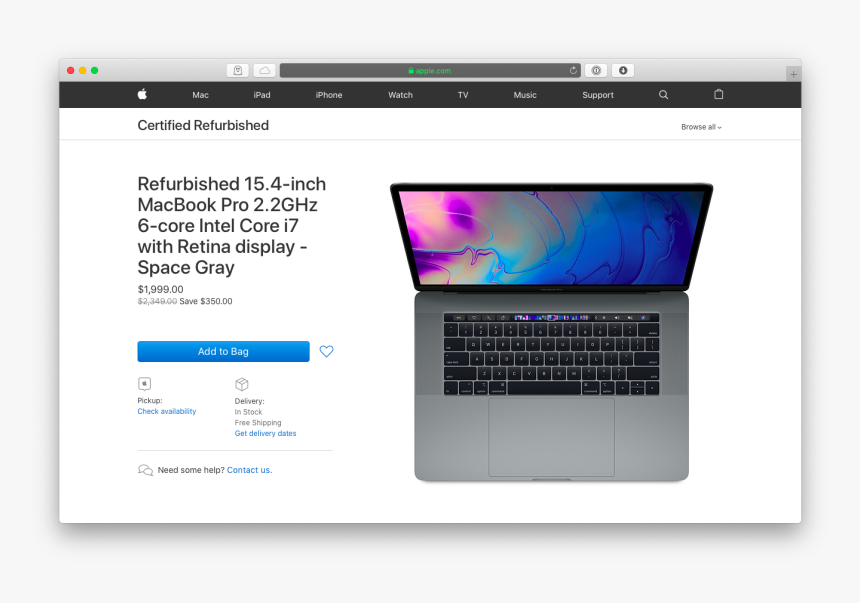The image showcases a screenshot set against a light gray background, centered in the middle. The screenshot features a gray header with three small round circles on the top left: red, yellow, and green, typically indicative of window controls. To the right of these circles, there's a search bar displaying the URL: "apple.com."

Below the header, the screen displays a black navigation bar from the Apple website. Starting from the left, there's a small Apple icon followed by the labels: Mac, iPad, iPhone, Watch, TV, Music, and Support.

The main content of the screenshot includes a large, color image of a MacBook Pro. To the left of this image, there is a section with text in large gray font. In the upper left corner, it reads "Certified Refurbished." Below that, it details the product description: "Refurbished 15.4-inch MacBook Pro 2.2 GHz 6-core Intel Core i7 with Retina display. Space Gray."

Beneath the product description, the price is listed as "$1,999," with the original price "$2,349" crossed out, indicating a saving of "$350." Below this information, there's a prominent blue action button that reads "Add to Bag."